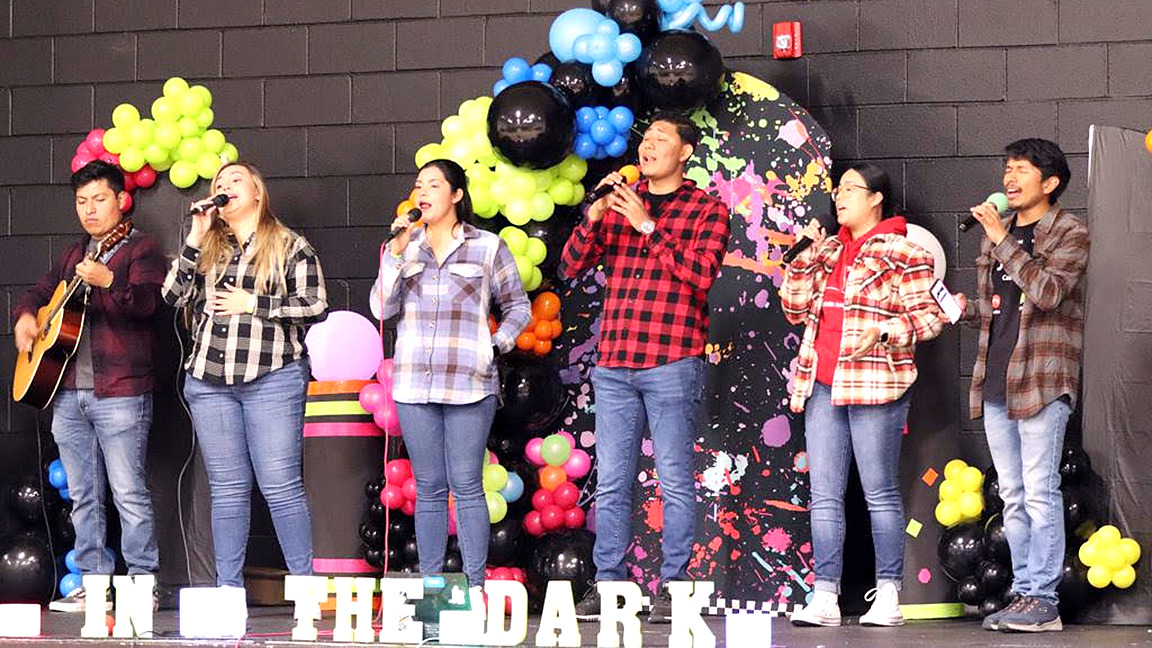In this rectangular photograph, we see a lively stage performance featuring a group of young people. The stage is elaborately decorated with vibrant balloons in shades of yellow, pink, and blue, positioned against a backdrop of rustic cinder blocks and a brown floor. From left to right, the performers are as follows: 

Firstly, a young man wearing a plaid shirt and denim jeans, skillfully playing an acoustic guitar. Next to him, a young woman with a microphone in hand is mid-song, her mouth open and her hand placed against her chest, conveying emotion as she sings. Following her is another young woman with dark brown hair, similarly dressed in a plaid shirt and denim jeans, also singing into a microphone. 

To her right stands a man in a red and black plaid shirt and denim jeans, passionately holding a microphone. Beside him, a young woman with black hair and glasses, dressed in a plaid shirt, jeans, and white sneakers, is also holding a microphone. Finally, on the far right, another young man is seen singing, dressed in a plaid shirt, brown denim pants, and blue sneakers. 

At the forefront of the stage, white block-style letters are prominently displayed in the dark, adding a final touch to this energetic and visually engaging scene.